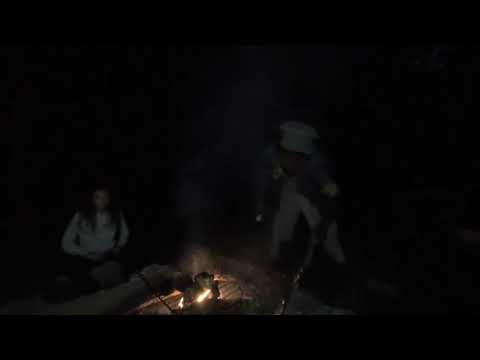In this very dark, nighttime photograph, two people are gathered around a small campfire that prominently illuminates the lower center of the image. On the left, a person with long hair is sitting down, wearing a white shirt. On the right, another person stands, dressed in white pants and a darker top, with a white helmet or similar headgear. The background is pitch black, rendering all the details beyond the immediate vicinity of the fire indiscernible. A metal tray or grill is visible over the fire, though it's unclear if there is anything on it. The glow of the campfire is the primary light source, casting the only significant illumination in the scene.